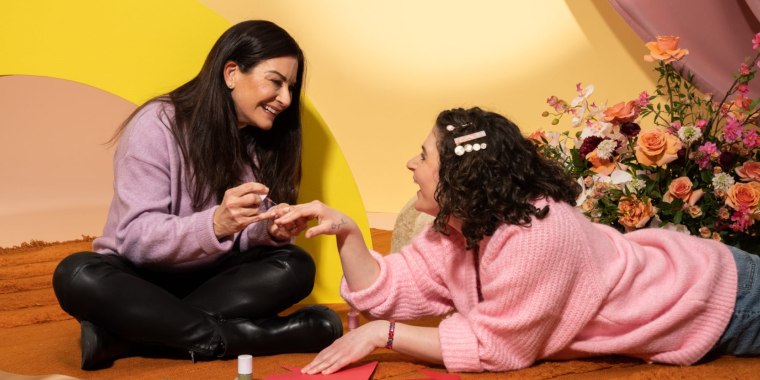The photograph captures a surreal, almost dreamlike scene featuring two women interacting on an orange carpet. The woman on the left is seated cross-legged, partially turned toward the viewer, and fully engaged with the woman on the right. She has long dark brown hair tucked behind her right ear and wears a light purple (plum-colored) sweater paired with black leather leggings and tall black boots. She is smiling warmly as she paints the nails of the woman on the right, holding a nail polish brush in one hand and the other woman's hand in the other.

The woman on the right is lying on her stomach, facing the woman on the left with a bright smile. She wears a pink sweater and blue jeans, her dark curly hair adorned with white barrettes. Her right hand is extended upward, receiving the nail polish treatment. Behind her is a large bouquet of flowers in shades of pink, peach, and white, accented with green foliage.

The background features an eclectic, abstract design with swaths of sunset colors—pinks and yellows. A prominent yellow arch is directly behind the seated woman, resembling an Escher staircase. This whimsical, kaleidoscopic setting gives the scene an almost hyperreal, cinematic quality reminiscent of shows like "Girls" or "Broad City," with an undercurrent of playful yet enigmatic tension in their smiles. Despite their mature appearance, the setting evokes the nostalgia of a teenage or preteen sleepover.